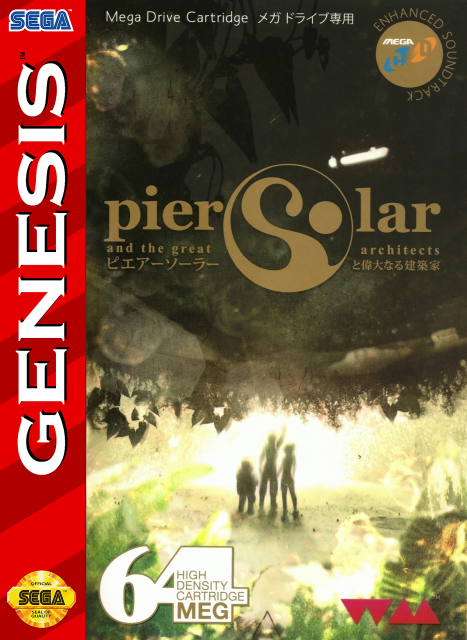This detailed color photograph depicts the cover of a Sega Genesis video game box. On the left side of the image, there is a distinctive red band with bold white text reading "Genesis." At the top of this band is the Sega logo in blue, while at the bottom, there is a gold medallion featuring the word "Sega" in black text. Across the top of the main body of the image, "Mega Drive Cartridge" is written in white text, and in the upper right-hand corner, there is an emblem bearing the words "Mega Drive."

Dominating the upper half of the main image, the words "Pier Solar" are prominently displayed in gold text, with the subtitle "and the Great Architects" underneath. Notably, the 'S' in "Solar" is stylized to resemble an earth. A watermark from Photobucket, reading "Protect More of Your Memories for Less," runs horizontally across the image. Below this strip, a forest scene features three human figures or silhouettes gazing up at what appears to be a distant rocket shooting into the sky. At the bottom of this scene, in large white text, the number "64" is displayed, with the phrase "High Density Cartridge Meg" inscribed within the numeral. Lastly, in the bottom right-hand corner, there are two upside-down and two right-side-up red triangles.